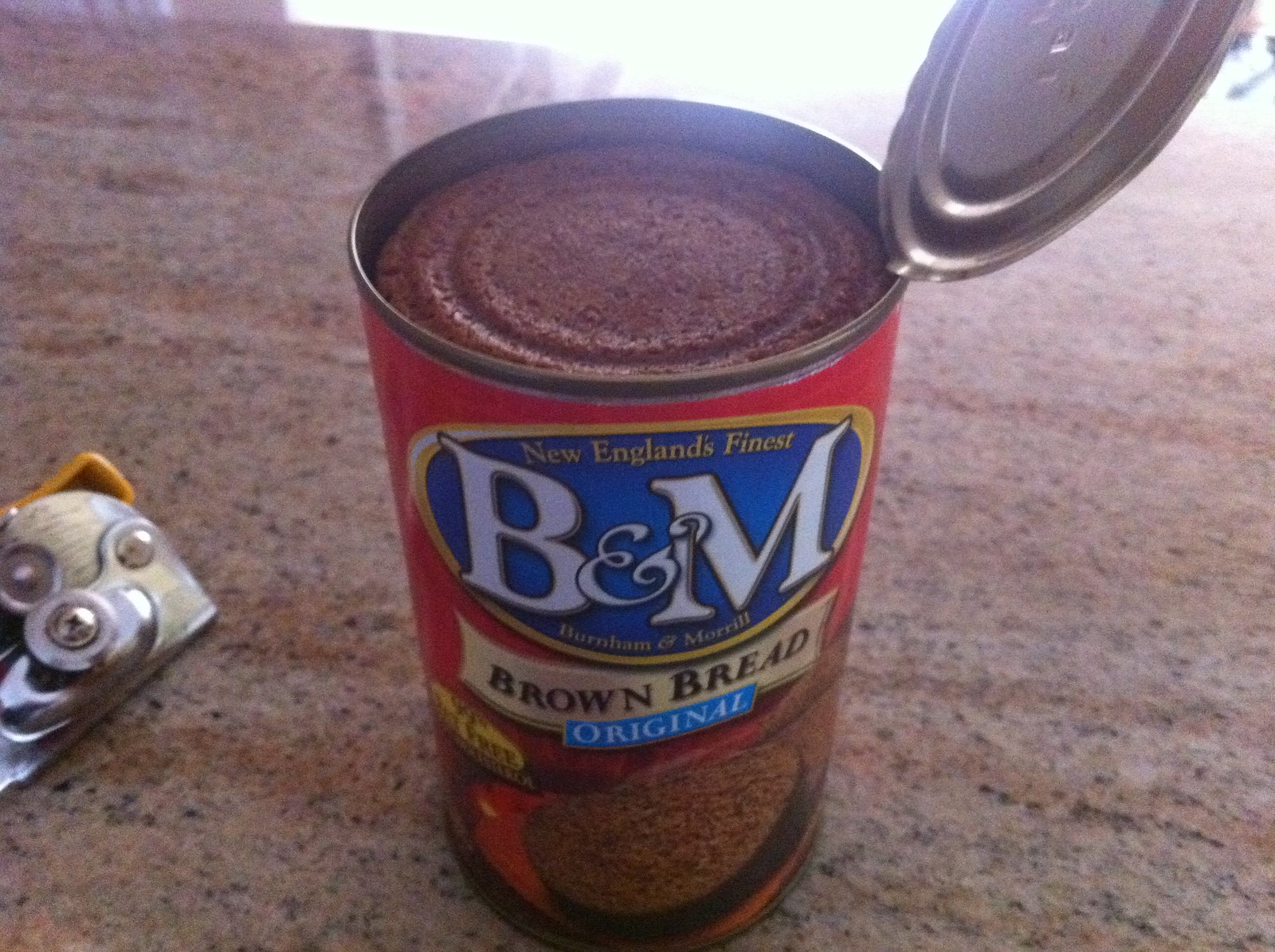The image displays an opened tin can of B&M brand brown bread, renowned as New England's finest. The can is sitting on a marble countertop, with a can opener lying to the left. The can opener is silver, featuring gears and a screw mechanism, with its top part visible on the right side of the photo. The can's lid is lifted, revealing the loaf of brown bread inside. The label on the tin can is prominently displayed, reading "B&M Original Brown Bread" and featuring the phrase "New England's Finest" along with the brand names B&M, Durham, and Morrell.